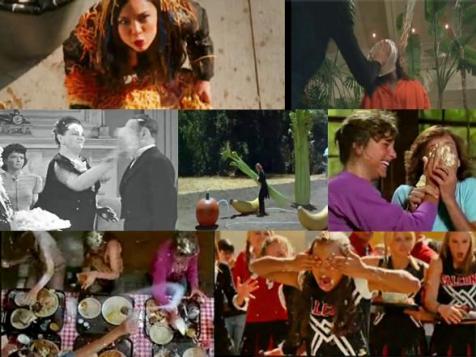The image is a collage consisting of seven distinct photographs. 

In the top-left corner, a woman in a black leather jacket sits in a parking lot, seemingly covered in spaghetti, looking upwards towards the camera. Next to her, another image features a woman in an orange shirt seated in front of a backdrop of lush plants, just as a man slams a pie into her face. 

The left-middle section of the collage displays a black and white photograph where a woman in black smashes a pie into the face of a man in a suit. The center photograph showcases a woman standing on a court surrounded by oversized fruit and vegetable sculptures, including a giant apple, bananas, and celery. 

To the right, another pie-smashing scene unfolds, this time with a woman in a purple sweatshirt applying a pie to a woman in a blue shirt. 

In the bottom-left corner, there’s a chaotic scene resembling a food fight, with someone spraying whipped cream or some form of white substance over a lunch table, splashing three people who are eating and now have food in their hair. The final image on the bottom-right portrays a girl, possibly a middle school cheerleader, wiping cream from her face with a group of girls standing behind her.